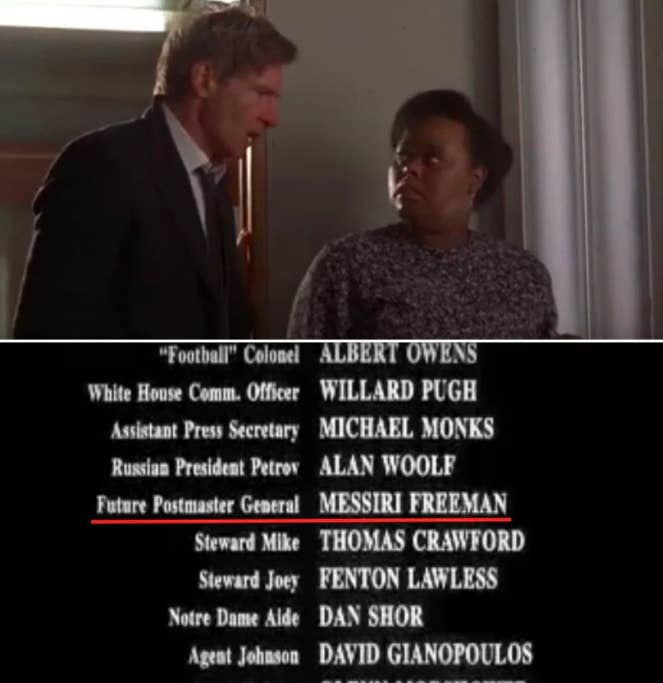In the image, the top half shows a scene from a movie featuring two actors. On the left is Harrison Ford, a white male with brown hair, wearing a black suit and tie, standing in a room with white walls and curtains. He is turned to the side and appears to be speaking to an African American woman beside him. The woman, dressed in a black and white speckled dress, looks up at Harrison Ford. The image is horizontally divided by a white line. 

The bottom half of the image displays the end credits of the movie against a black background, with white text listing various characters and actors. Some notable mentions include "Football Colonel Albert Owens," "White House Comm Officer Willard Pugh," "Assistant Press Secretary Michael Monks," "Russian President Petrov Alan Wolf," "Future Postmaster General Massiri Freeman," "Steward Mike Thomas Crawford," "Steward Joey Fenton Lawless," "Notre Dame aide Dan Shore," and "Agent Johnson David Gianopoulos." The character names are written in mixed-case letters, while the actors' names are in all-uppercase letters. Additionally, there is a red line underlining the words "Future Postmaster General, Messiri Freeman."